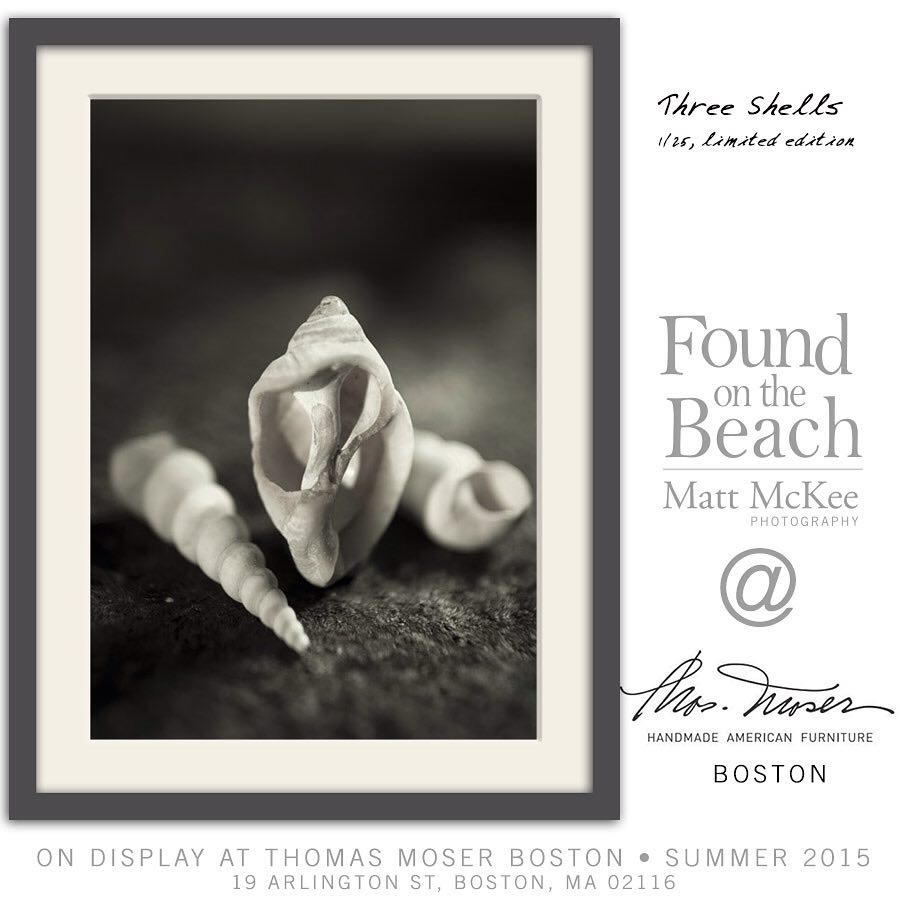The image is a black and white photograph of three seashells, displayed inside a gray picture frame with a white inner border. The seashells, arranged next to each other in a spiral pattern, rest on a rough gray surface. The central shell is oval-shaped, showcasing its white and gray crest and its intricately detailed interior. To the right of the picture frame, there's handwritten text stating "three shells," marked as a "1/25 limited edition." Below this, in various shades of gray text, it reads "found on the beach," attributed to "Matt McKee photography." Further down, there is a note: "on display at Thomas Moser, Boston, summer 2015," followed by the address "19 Arlington Street, Boston, MA 02116." An indistinct, scripted signature is also present, along with a mention of "Handmade American furniture."